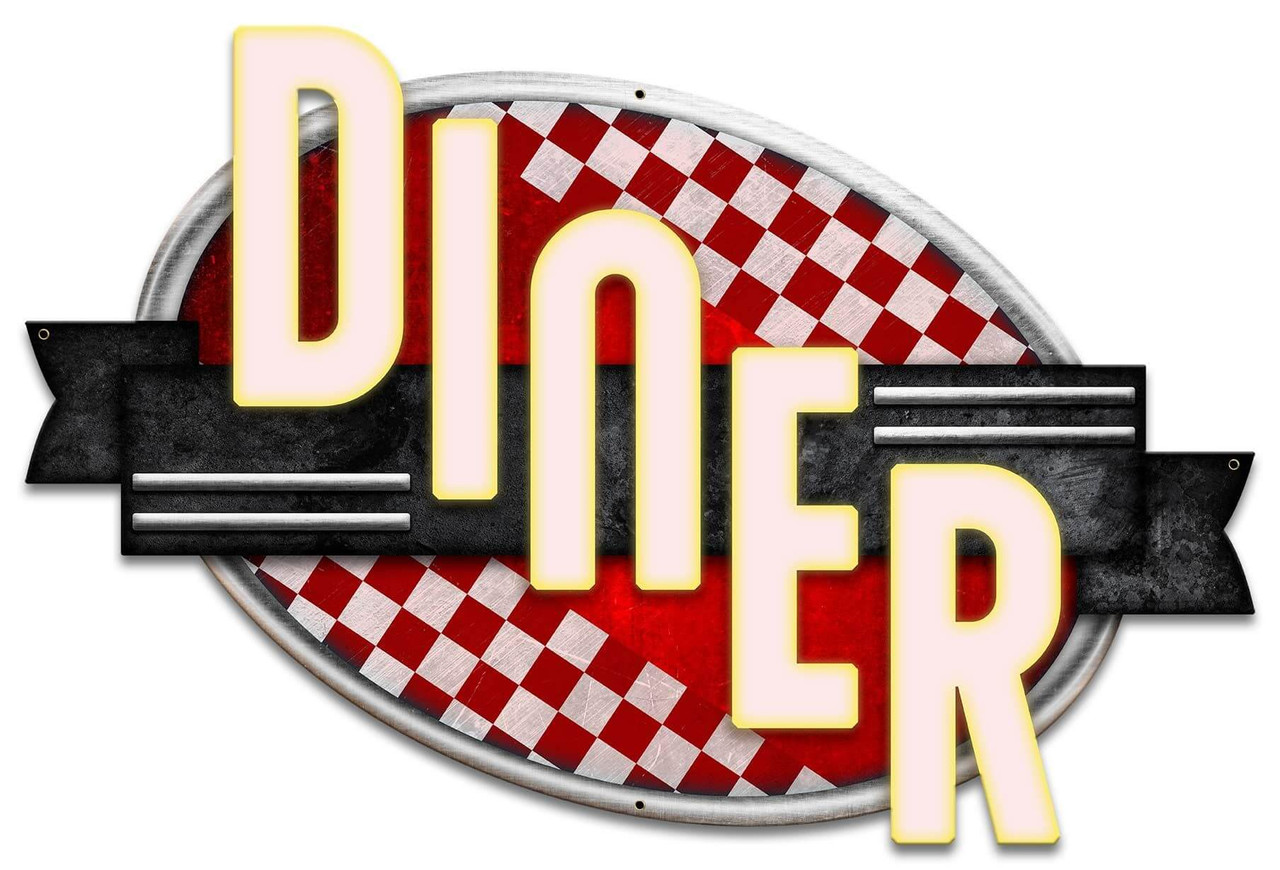The logo for the diner is designed in a retro 1950s style, embodying the classic aesthetic of the era. The word "DINER" is prominently displayed in large, white letters with a yellow outline, stacked vertically at an angle from the top left (D) to the bottom right (R). These letters sit atop a black, horizontal banner that features chrome pinstriping on either side, contributing to a chalkboard-like texture.

Behind the banner, a visually striking oval background anchors the design. This oval is oriented in the same diagonal direction as the letters, featuring a red stripe running through its center. Surrounding this stripe is a red and white checkered pattern, reminiscent of vintage diner decor. The entire oval is framed with a chrome border, enhancing its retro appeal.

The logo exudes the vibrant, nostalgic charm of a classic neon sign, making it an ideal emblem for a diner or a related eating establishment.